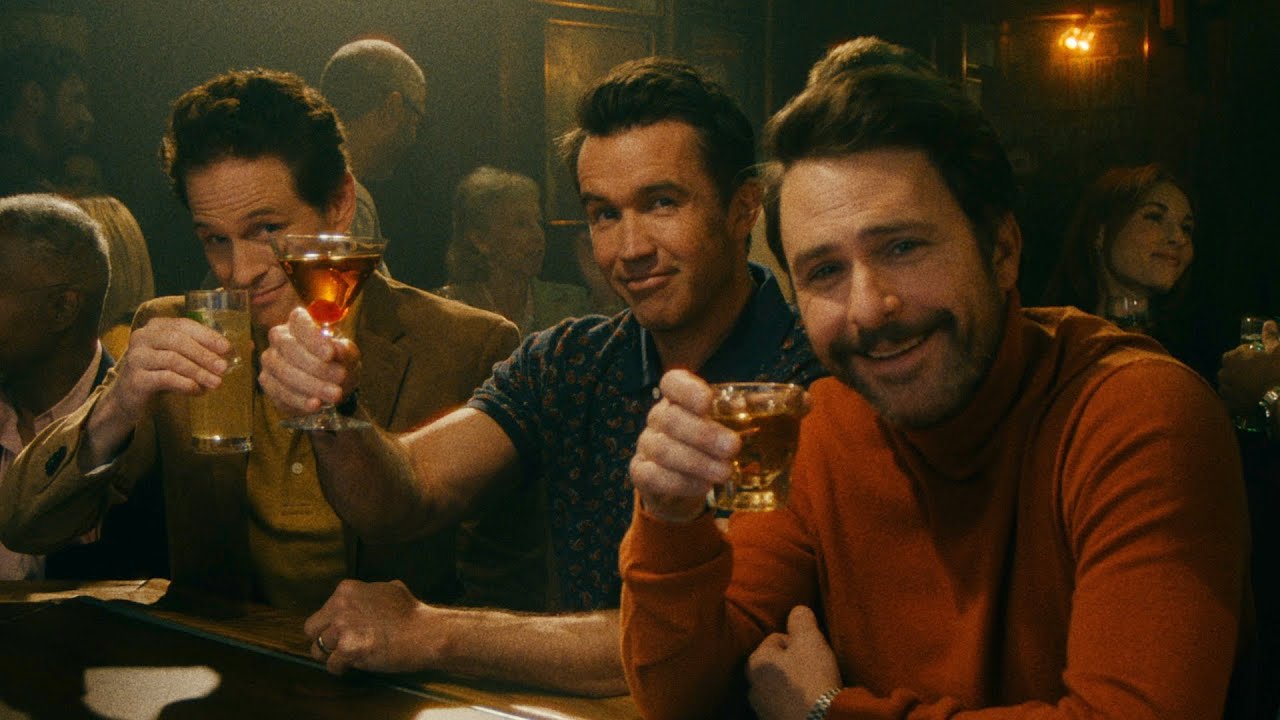In this up-close photo of three men enjoying cocktails at a bar, all are smiling and gazing intently at the camera, each holding a drink in their right hand in a celebratory toast. The lighting is focused on the trio, making their features stand out against the dimly lit bar background where other patrons can be seen in muted conversation. 

On the left is a gentleman with curly, poofy brown hair and a flawless smile. He’s wearing a mustard-colored casual shirt paired with a brown jacket. He holds a tall Collins glass filled with a yellow, pineapple-like liquid. 

The middle gentleman, bearing a close resemblance to Burt Reynolds, sports a navy blue, short-sleeved polo with a pattern on it. He holds a martini glass containing a brown liquid, likely a Manhattan, with a cherry at the bottom.

The man on the right, identified as Charlie Day, dressed in a rust-colored, long-sleeved turtleneck, has a mustache and brown hair. He holds a small shot glass filled with a dark liquor, possibly whiskey. 

All three men share similar dark, wavy short hair and exude a warm, convivial vibe. The entire scene is bathed in a warm filter, enhancing the cozy atmosphere of the bar.